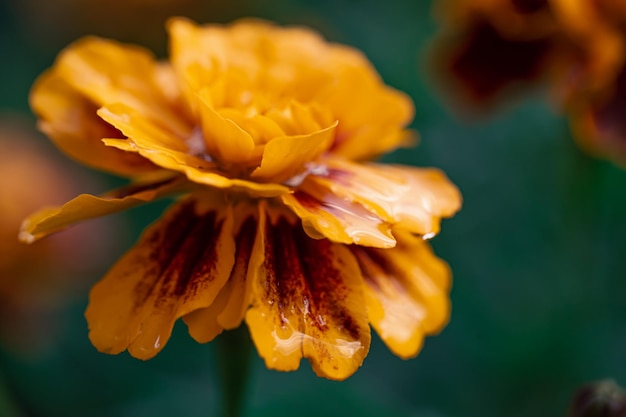The high-resolution photograph captures an intricate, super zoomed-in view of a single flower in full bloom, predominantly displaying its vivid, mustard-yellow petals with a rich, dark red center that fades into orange and hints of black. The freshly rained-upon petals glisten with droplets of water, giving them a waxy appearance as they drip down onto the ground. The focus of the image is entirely on the bloom, as indicated by the sharply detailed petals and the blurred, teal-blue to hazy green background, where three other flowers are barely discernible. The blurred stalk of the flower contributes to the overall sense of depth, emphasizing the vibrant bloom set against the contrasting backdrop.